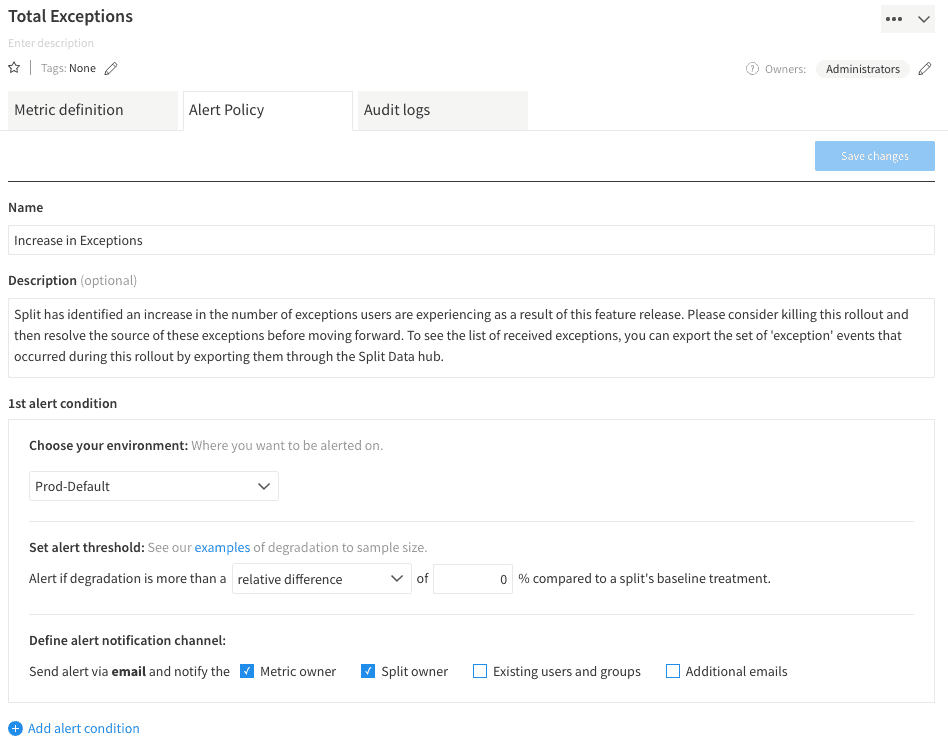The image displays a user interface for configuring alert policies. At the top, under the header "Total Exceptions," there is a light-gray placeholder text that reads, "Enter description." 

The interface is segmented into three distinct sections: "Alert Policy" in focus, with "Metric Definition" to the left and "Selection for Audit Logs" to the right. A black divider line separates the header from the main content.

Immediately to the right and atop the black divider line is a button labeled "Save Changes."

Below the divider line on the left, there is a label "Name," next to which is a text input box containing the text "Increase in Exceptions." Beneath this, there is a light-gray, optional description field with the placeholder text, "(Optional)". Inside the description field, it states: "Split has identified an increase in the number of exceptions users are experiencing as a result of this feature release." The description further mentions the potential of terminating the project.

The following section has the bold title "First Alert Condition." This area includes instructions to "Choose your environment where you want to be alerted on," with a drop-down menu that defaults to "Prod."

Next is the "Set Alert Threshold" section, followed by the "Define Alert Notification Channel" section at the bottom of the page. Here, notifications can be sent via email alerts with four checkboxes available: "Metric Owner" and "Split Owner" are checked, while "Existing Users and Groups" and "Additional Emails" are outlined in blue but unchecked.